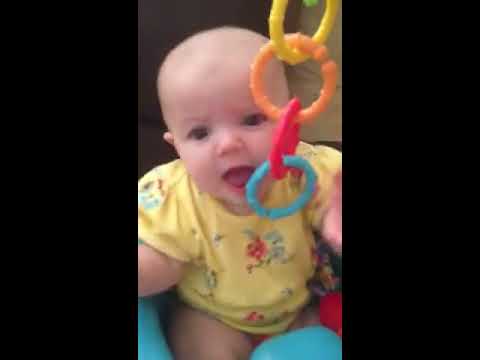The photograph, seemingly taken from a smartphone and vertically cropped, centers on an infant, possibly around 4 to 5 months old, devoid of hair and adorned in a yellow onesie decorated with red, blue, and green floral patterns. The baby, seated in what appears to be a light teal-blue baby seat or car seat with visible straps, gazes towards the camera with an open mouth, as if smiling and attempting to grasp a set of interconnected plastic rings hanging in front of them. These rings, colored in sequence from top to bottom as yellow, orange, red, and light blue, dangle enticingly near the infant's mouth. The image is bordered by black vertical rectangular areas, emphasizing the vibrant and central details of the baby and the playful rings, with a blurred off-brown wall faintly noticeable in the background.